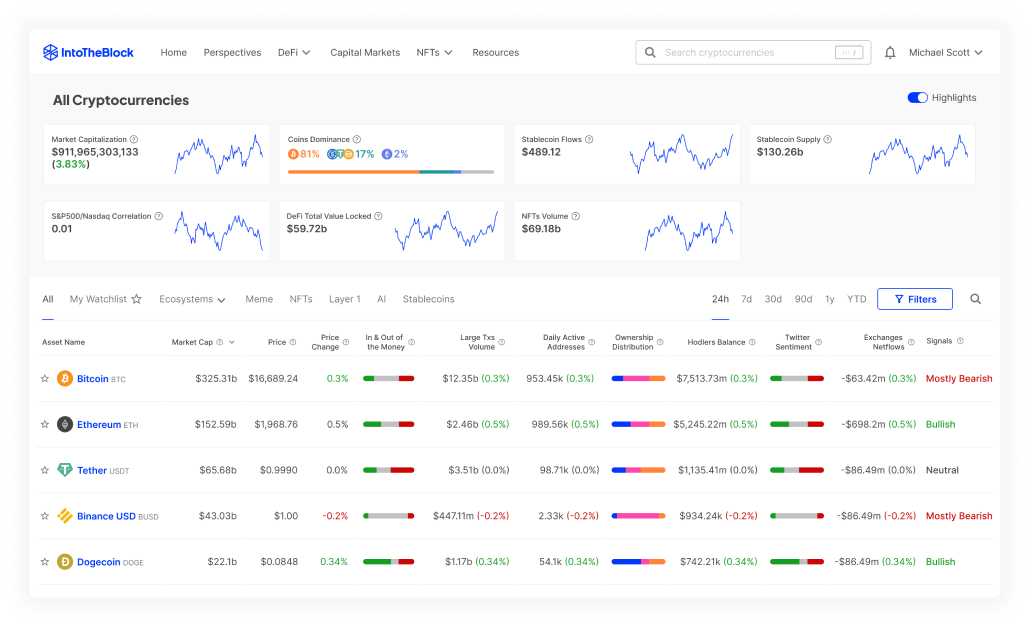The image depicts a detailed webpage displayed on a computer screen, specifically focused on cryptocurrency and financial markets. At the top of the page, the header bar features a section labeled "Into the Block," followed by several navigation tabs: "Home," "Perspectives," "Defy," with a down arrow indicating a dropdown menu, "Capital Markets," "NFTs," also with a down arrow for additional options, and "Resources." On the far right of the header bar, there is a small search engine box accompanied by a magnifying glass icon, a bell icon representing notifications, and a profile section with the name "Michael Scott" and a down arrow suggesting a dropdown menu.

On the far right side of the header, the term "All Cryptocurrencies" is displayed. Just below the navigation, the interface shows "Highlights" turned on. Below this, there is a section labeled "Market Capitalizations," followed by "Coins Dominus," "Stable Coin Flows," each accompanied by a graph showing fluctuating data.

To the side, there are various financial metrics accompanied by graphs: "Stable Coin Supply," "S&P 500 NASDAQ Correlation," with a graph beside it, "DeFi Total Value Locked," and "NFTs Volume," all with corresponding numerical data beneath.

In the middle to the lower section of the page, the interface includes categories such as "All My Watchlist," with subcategories like "Ecosystems," "Mean," "NFTs," "Layer 1 AI Stable Coins," and various timeframes: "24 Hours," "7 Days," "30 Days," "90 Days," "1 Year," "YTD (Year to Date)." There is also a filter box with a magnifying glass icon for refined searches.

Below these settings, the webpage lists asset names such as "Bitcoin," "Ethereum," "Tether," "Binance USD," and "Dogecoin," each accompanied by corresponding statistical data to the right.